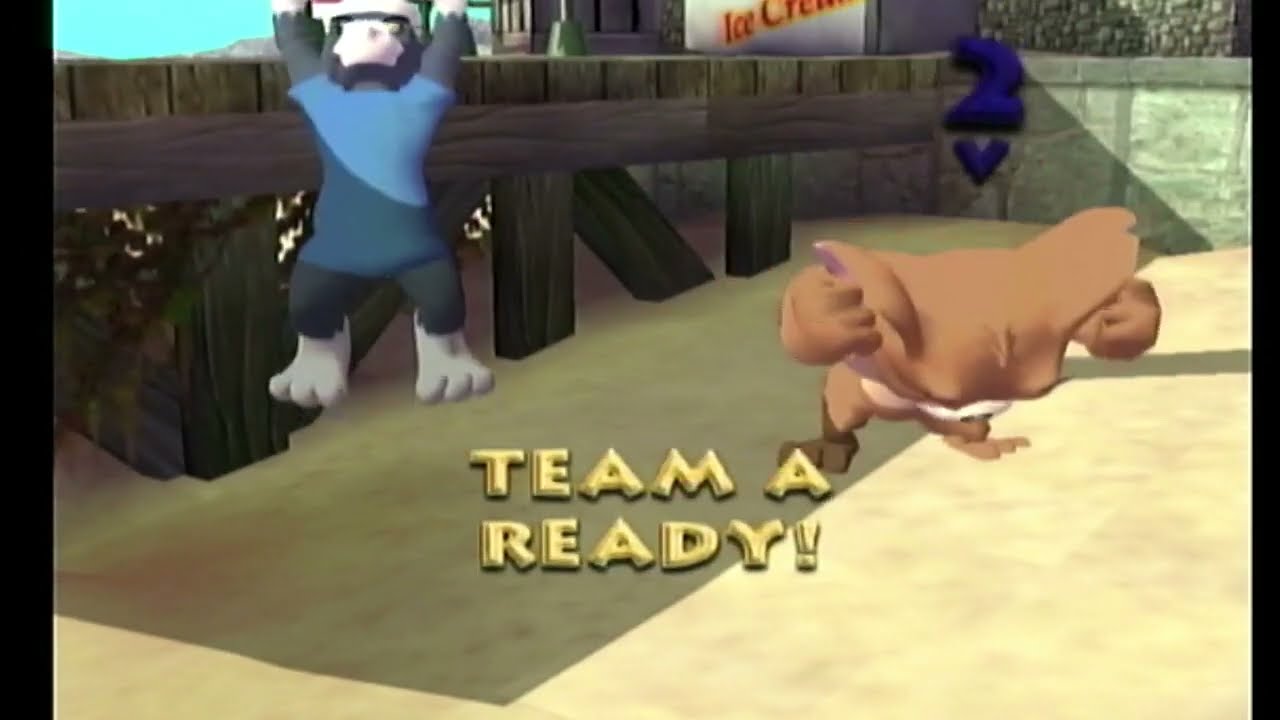The image is a digital screenshot from a video game featuring an outdoor scene, likely an arena or competitive setting. In the center-right of the image, there is a brown character with large ears, hunched over with its hands up by its ears, possibly resembling a cartoonish animal like an owl or bear. This character has big brown feet and a white snout. To the left of this character stands another character with dog-shaped white feet, wearing a two-tone blue top, and with its arms raised triumphantly over its head, suggesting a victorious pose. The background includes a wooden platform-like structure and possibly a pier, with sand and a wall further behind. Above the hunched-over brown character, the number '2' accompanied by an arrow is visible. The text "Team A Ready!" is prominently displayed at the bottom of the image. The overall color scheme includes shades of brown, tan, beige, dark gray, reddish gray, blue, dark blue, black, and red. The style is digital art typical of video game graphics.